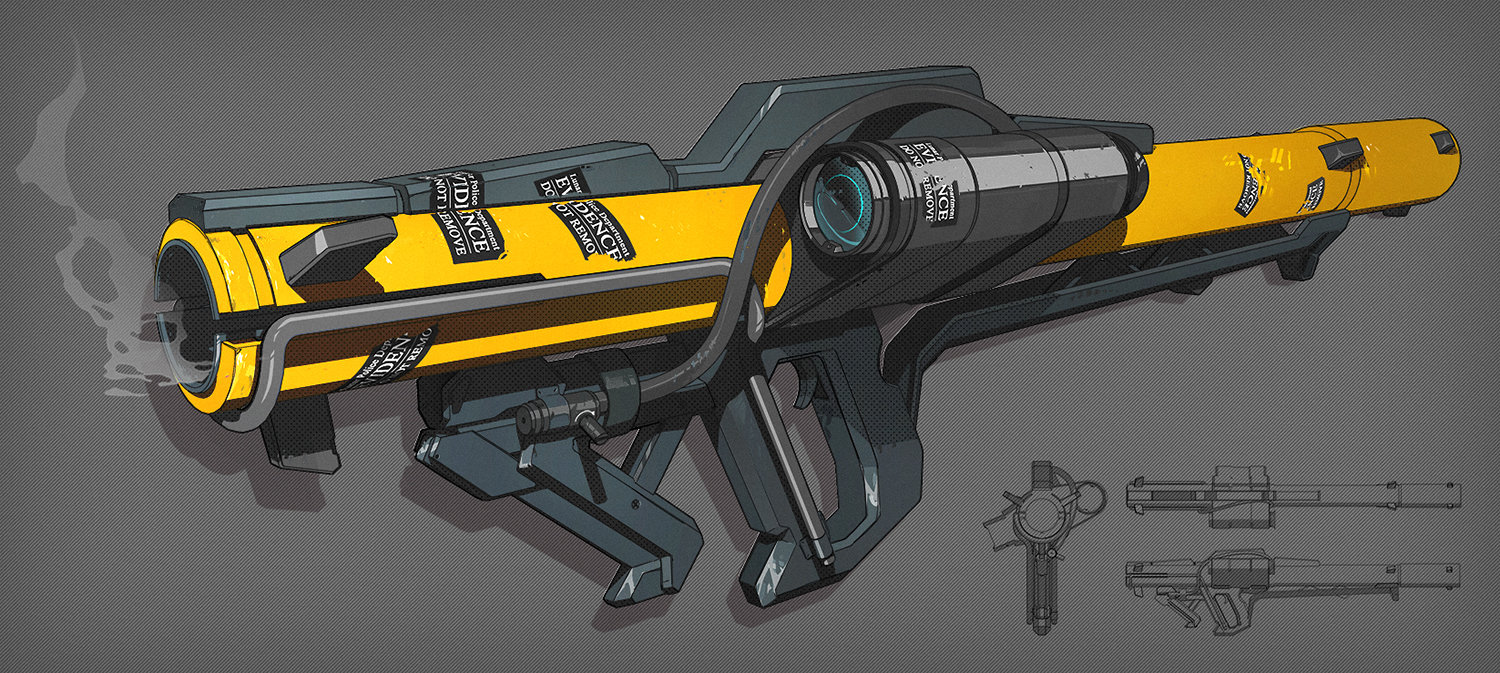This animated image, set against a medium gray background in landscape orientation, features a detailed prototype of a high-powered weapon resembling a bazooka. The weapon has a thick, straight yellow barrel with white smoke emanating from its end and is adorned with black and white "law enforcement evidence" stickers. A sturdy black handle with an integrated trigger mechanism is positioned below the barrel, accompanied by a gray brace for support. Additionally, a black scope is mounted on one side, complemented by a gray rubber tube connecting it to the area beneath the barrel. Above the barrel, there is a thick, shiny gray fin. In the lower right corner, three detailed diagrams are presented, illustrating the weapon's view from the top, side, and down the barrel. The entire weapon design is rendered in a cohesive color scheme of yellow, black, and gray.